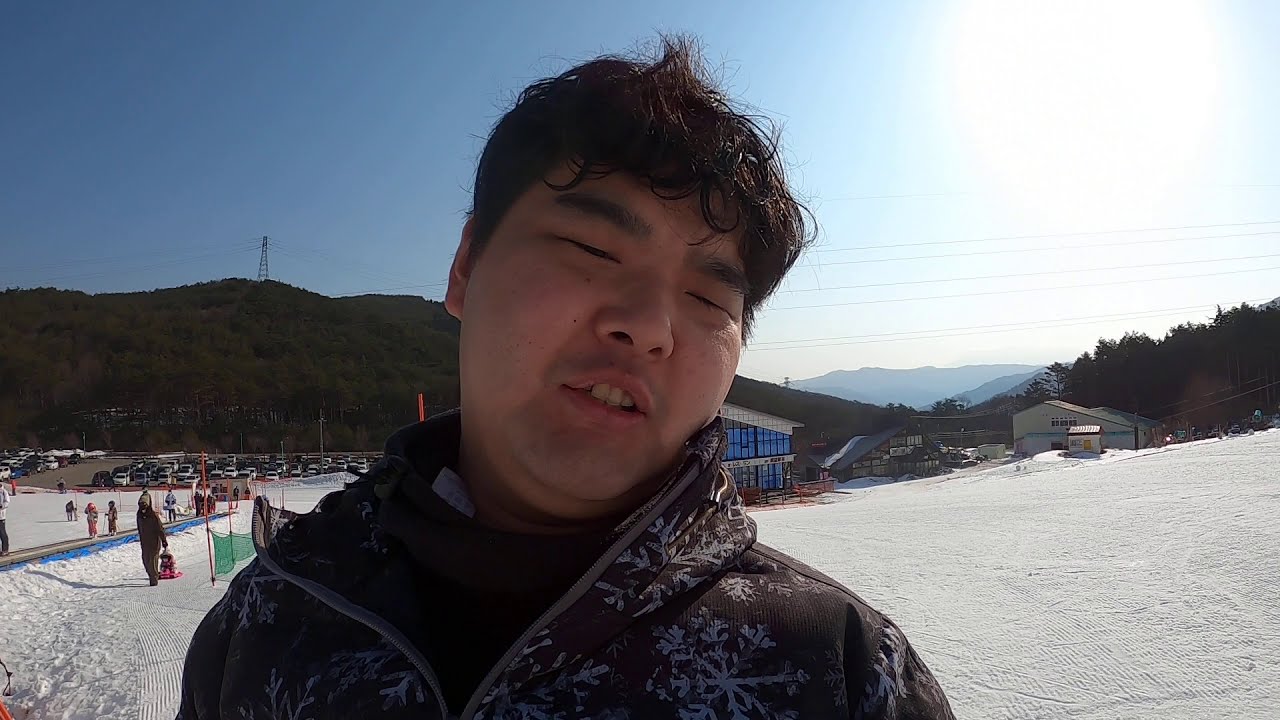In the foreground of the image, an Asian man with short black hair and dark eyebrows stands on a snow-covered ski slope, looking directly at the camera. He has small, squinted eyes, likely due to the bright sunlight indicating a clear, blue sky without any clouds. The man, who has a round face with a slightly open mouth, is dressed in a black or dark gray snow jacket adorned with large snowflake designs. His head is tilted slightly to the side as if he is in mid-conversation.

Surrounding him on this bright, sunny day are several other individuals dressed in heavy winter clothing, some walking and others possibly sledding, primarily on the left side of the frame. In the mid-ground, a sprawling parking lot is visible, filled with numerous cars, suggesting the place is a popular recreational area. Behind the parking lot, there's a green mountain devoid of snow, as well as some buildings that might include a lodge or ski-related structures. To the far right, there appears to be a ski lift area, though it is distant and somewhat indistinct. Additionally, there are power line towers in the background, adding to the sense of a well-developed ski resort.